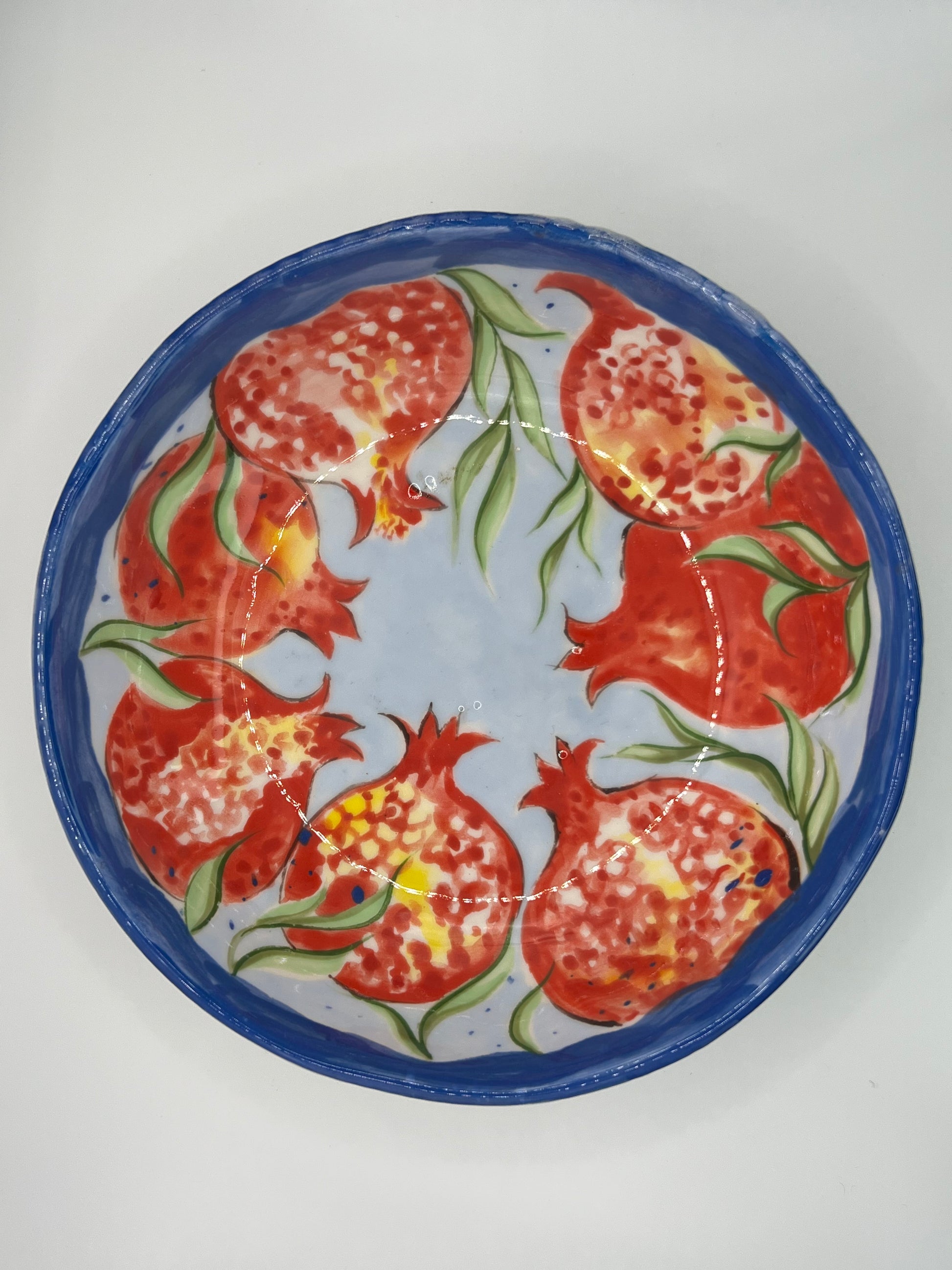This image features a vibrant, hand-painted ceramic bowl with a strikingly detailed design. The bowl's rim is a deep royal blue, while the inner surface is adorned with a rich display of red-colored pomegranates interspersed with thin green leaves in varying shades. Among the pomegranates, there are hints of yellow and occasional blue dots that add to the complexity of the design. Some pomegranates appear intact, while others seem cut open, adding to the realistic portrayal. The bowl sits on a white to gray surface and has a shiny center, likely reflecting light. The craftsmanship suggests it is handmade, with the meticulous painting style and careful placement of elements contributing to its elaborate aesthetic.